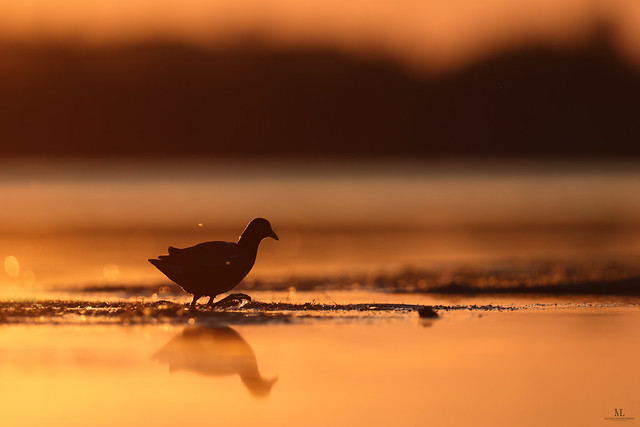In the serene outdoor setting of either a sunset or sunrise, the scene is awash with an enchanting orange hue. There's a small bird, possibly a duck, standing solemnly on a muddy patch that slightly protrudes from the tranquil water. The bird is silhouetted against the vibrant sky, facing right in profile, showcasing its beak, wings, and feet distinctively. The water surrounding it is smooth and mirror-like, reflecting the bird perfectly without a single ripple to distort the image.

In the distance, a dark mass, likely trees, extends across the horizon, partially blurred amidst the glowing orange backdrop. Below this, a faint hint of blue and white streaks runs horizontally, suggesting another body of water or perhaps a distant landform. The sunlight appears to sparkle on the water's surface, creating lighter, glistening patches reminiscent of scattered drops. The overall scene portrays a calm yet vivid depiction of nature, blending the stark silhouette of the bird with the soft, glowing colors of the dawn or dusk.